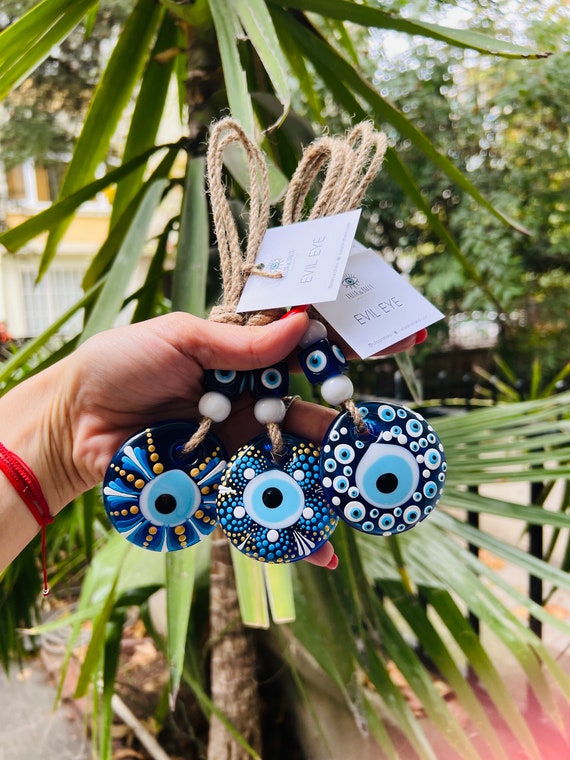In the image, a fair-skinned woman with red painted nails and wearing a red bracelet is holding up three intricately designed evil eye decorations, each attached to a rope. The decorations are pendants crafted to look like mandalas, combining circular and floral patterns with vibrant blue, black, and white colors. Resembling peacock feathers or water droplets, these pieces feature an 'eye' design in the center, surrounded by detailed dot motifs. Additionally, each ornament has tags still attached, indicating they are for sale. The woman's left hand showcases these artisanal items against an outdoor backdrop with visible tree branches and green leaves, suggesting a natural, possibly island-like, setting.